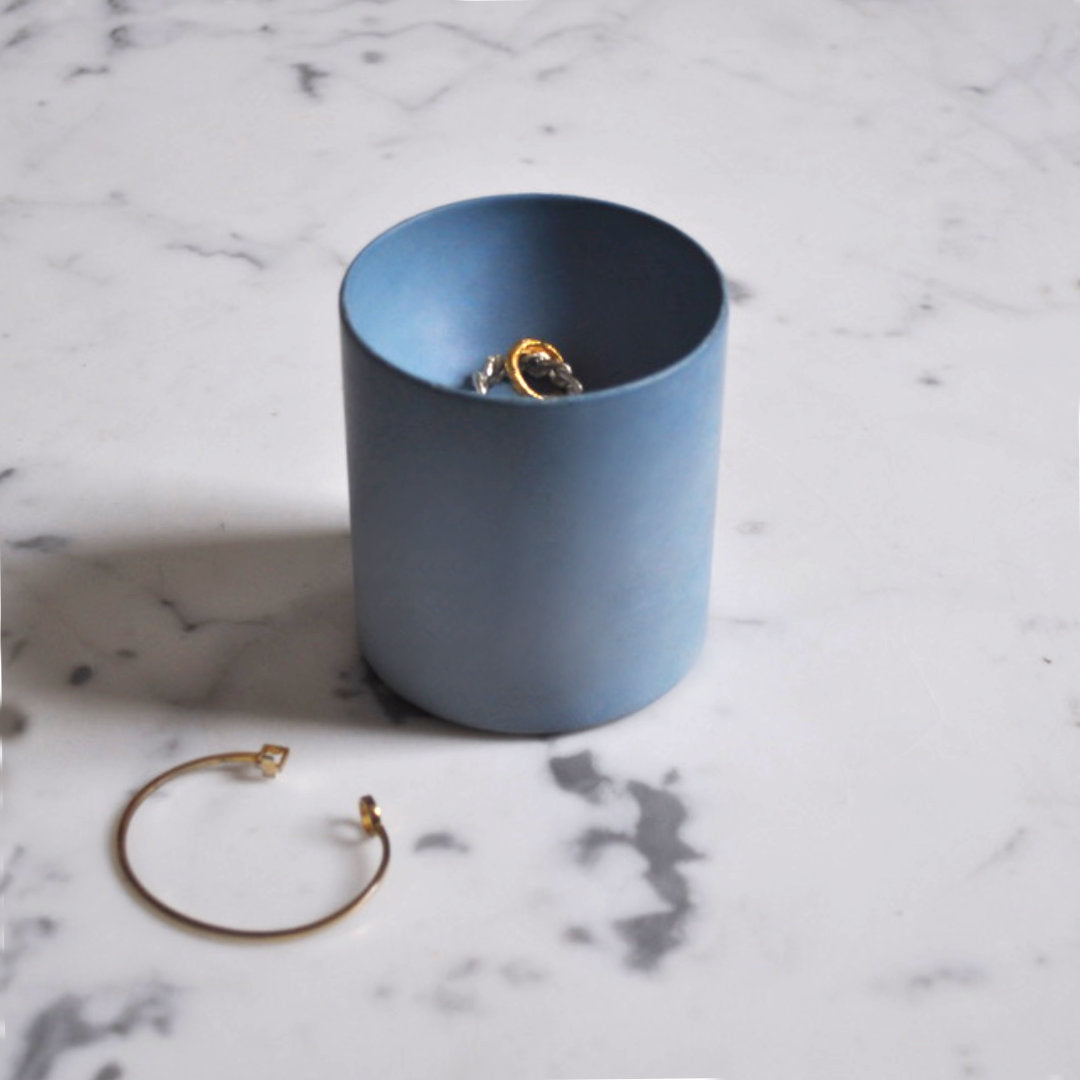In this square-cropped, close-up image taken at a 45-degree angle, a light blue cup sits at the center of a white marble or quartz countertop that features faint dark gray patches. Inside this cup, which stands about two to three inches tall, lies a couple of pieces of jewelry: a small silver piece and a round, bright gold item that resembles a small hoop earring. Outside the cup, on the left-hand side, rests a large gold hoop earring, approximately one and a half to two inches across, laying open on the counter. Additionally, an open gold cuff bangle is situated in the lower left corner of the image. The lighting, coming from the right side, casts a shadow to the left of the cup, highlighting the polished and detailed appearance of the scene.